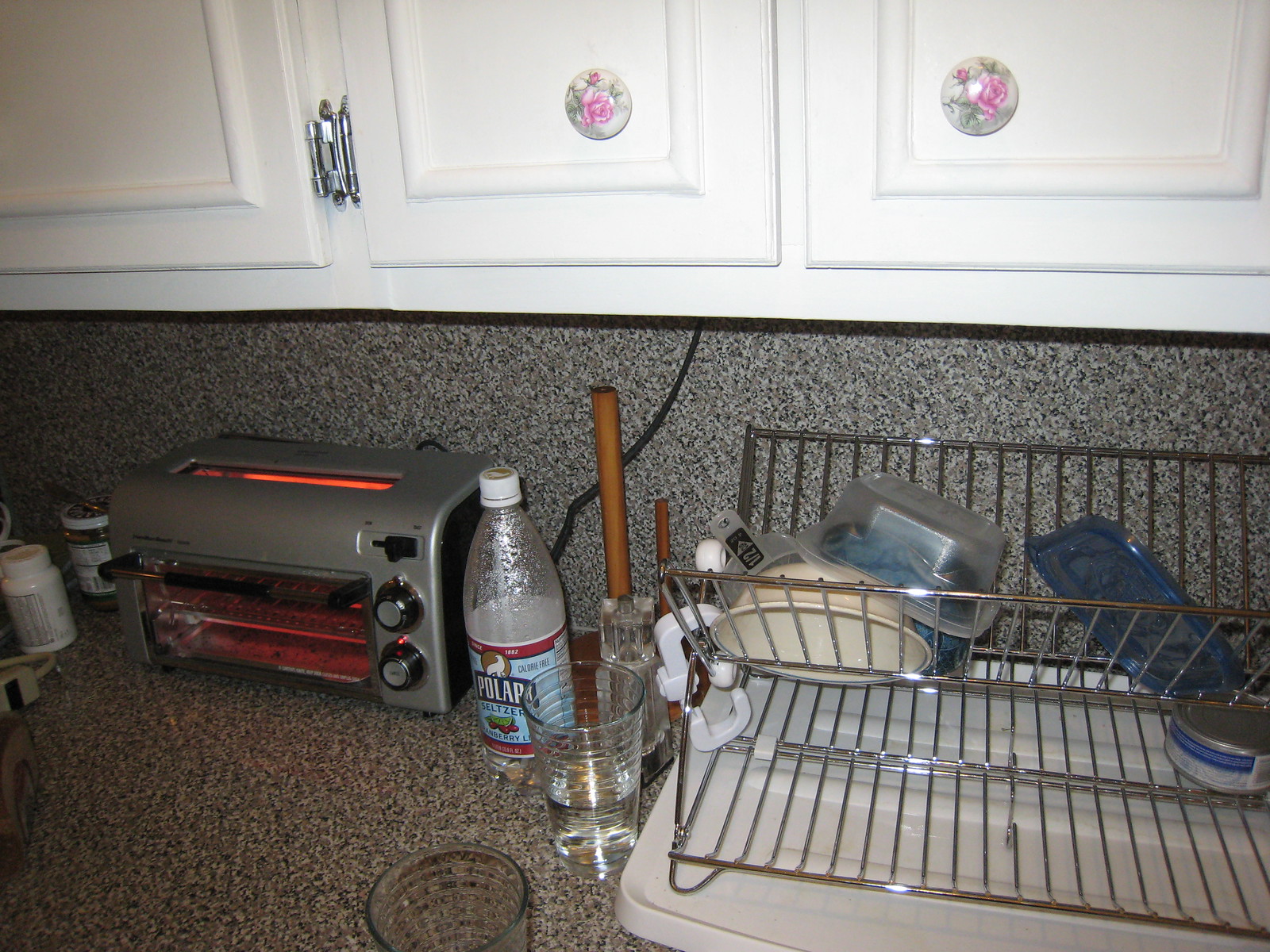In this detailed image of a kitchen, a granite stone-like backsplash accentuates the inviting space. The kitchen counter, spanning the width of the photograph, hosts an array of everyday items. On the far right, a white tray sits beneath a drain board, hosting an assortment of plastic containers and a bowl. Moving left, three glasses are lined up, with the middle one filled halfway with water. Further down, a 16-ounce Polar Seltzer bottle, resembling a half-liter size, stands next to a toaster oven glowing with red light, toasting a couple of slices of bread. Adjacent to the toaster oven, a couple of small bottles—potentially containing vitamins or over-the-counter medications—are neatly placed. Above this countertop, three cabinet doors, adorned with silver hinges and knobs featuring pink flowers and green leaves, lend a touch of charm to the kitchen's overall aesthetic.